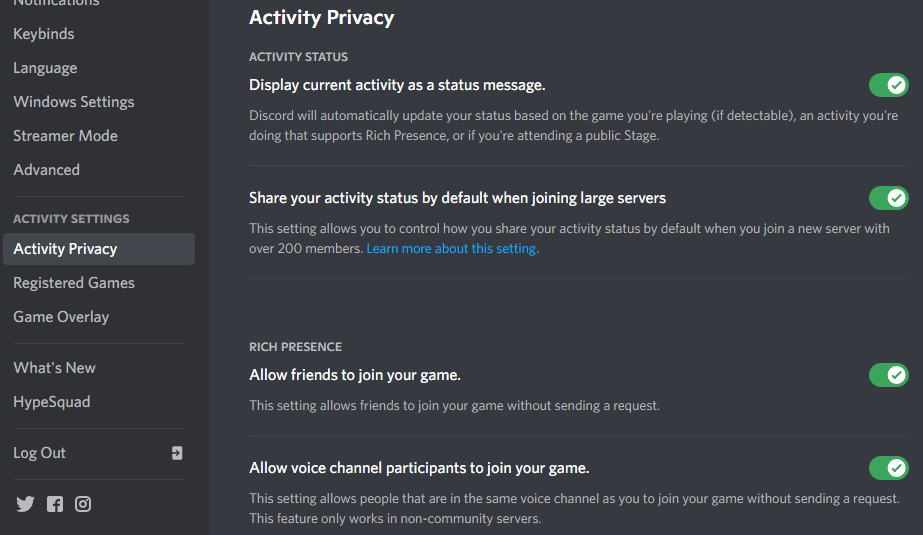The image showcases a user interface from the Discord application. The background is divided into two sections. The right side features a dark slate gray backdrop, while the left side is backed with black and contains a fully left-justified navigation menu. The navigation menu items listed are: 

- Keybinds
- Language
- Windows Settings
- Streamer Mode
- Advanced
- Activity Settings (in capital letters)
- Activity Privacy
- Registered Games
- Game Overlay
- What's New
- Hypesquad
- Logout
- Twitter
- Facebook 
- Instagram

The right side of the screen focuses on the "Activity Privacy" settings. The first option, "Activity Status," reads: "Display current activity as a status message. Discord will automatically update your status based on the game you are playing if detectable and if the activity supports Rich Presence or if you're attending a public stage." This option is toggled on and displayed in green. A note below explains that the user's shared activity status will default when joining large servers with over 200 members, providing users with more control over how their activity status is shared by default.

Further down, another setting labeled "Rich Presence" reads: "Allow friends to join your game. This setting allows friends to join your game without sending a request," which is currently toggled off. 

A "Learn more about this setting" link is highlighted in blue, offering additional information for users who require more context.